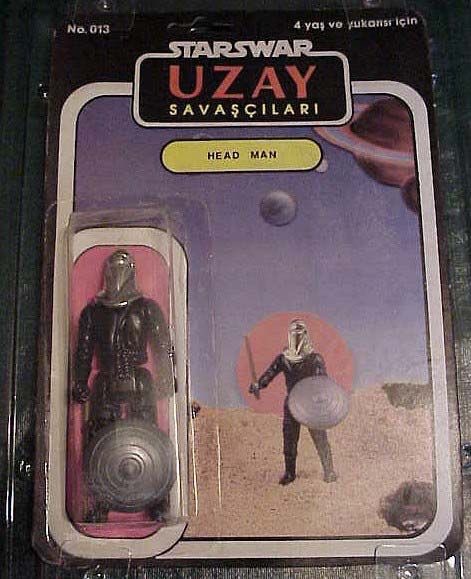The image features the packaging of a toy figurine that is a knockoff of the Star Wars franchise, labeled as "Stars War." At the top of the packaging, "Stars War" is written in white font, accompanied by another word, "Savas Kilari," both set in a font reminiscent of the original Star Wars logo. Below this, the name "Use A" appears in red. The top-left corner indicates the product number "NO. 013," while the top-right displays a number "4" followed by additional text in an unknown language. The packaging includes a predominately black background with an illustration of the character in the center, depicted standing on a sandy surface with a rising sun and planets resembling Saturn in the sky. The character wears a black uniform with a silver helmet and a shield. The bottom left of the packaging shows the actual toy encased in plastic, featuring the same black armor, a medieval-style silver helmet, and a silver shield with a spike. Additionally, a yellow oval icon with a black border and the word "Headman" in the center is present below the character.